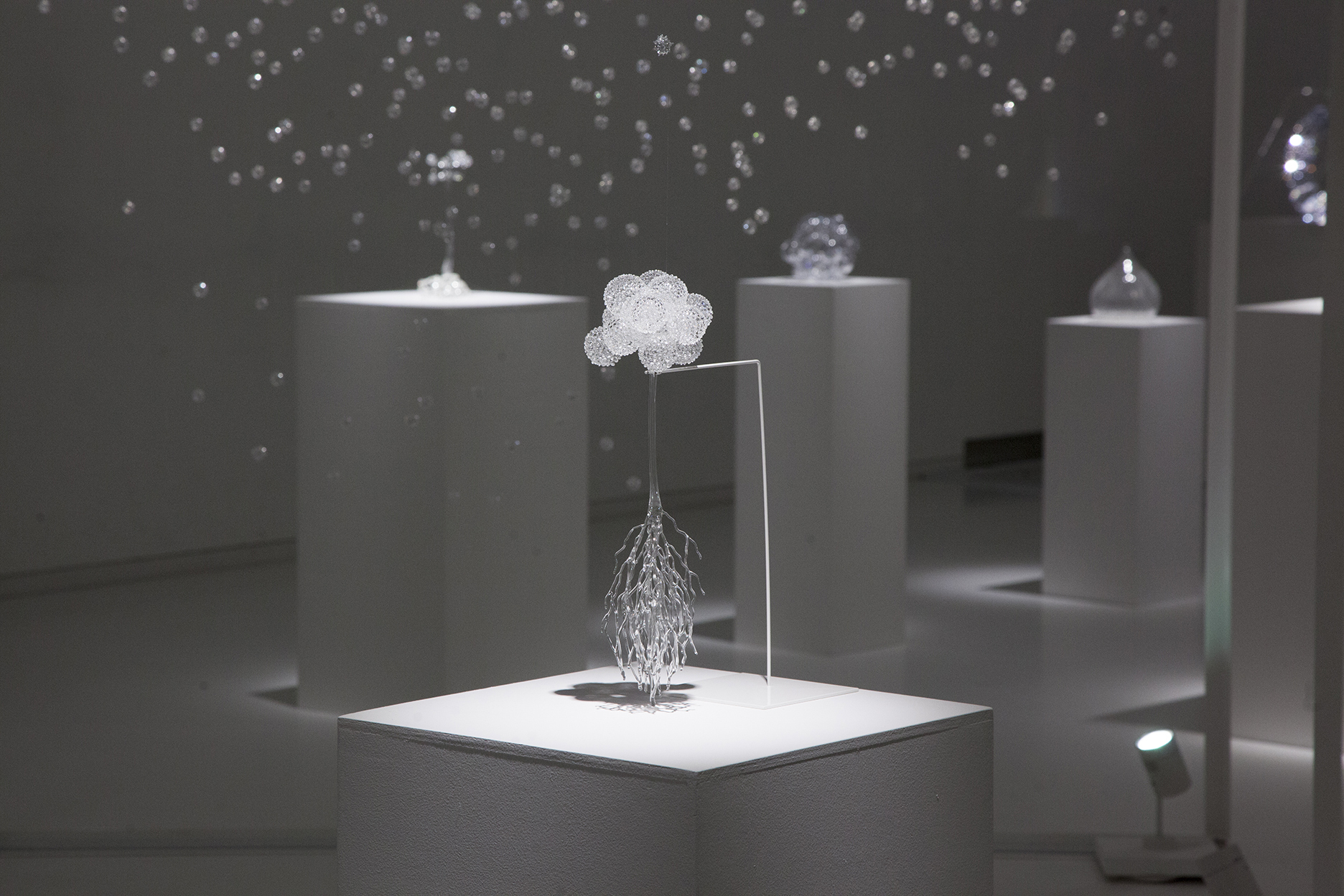The black and white photograph depicts an artistic display scene, likely in a museum or art gallery setting. The entire room is composed of varying shades of gray, from darker gray to charcoal, with certain areas so light they almost appear white. Central to the image are various square pillars of varying heights, each crowned with an ornamental crystalline structure that exudes a non-utilitarian essence. The most prominent pillar is in the foreground, shorter and well-lit, indicating overhead lighting. From the back of this low pillar, a wire arches forward, holding a cluster of tiny, luminous orbs. Descending from this cluster is a string adorned with fibrous, translucent tendrils, resembling roots or delicate glass strands, which hover gracefully above the pillar’s surface.

In the background, additional similar structures are visible, mounted atop tall white boxes, though their details are blurred and indistinct. The room also exhibits floating bubbles or light reflections, enhancing the ethereal atmosphere. Together, these elements create an intricate and artsy visual ensemble, with clusters of glass spheres and root-like tendrils that resonate with both natural and abstract qualities.